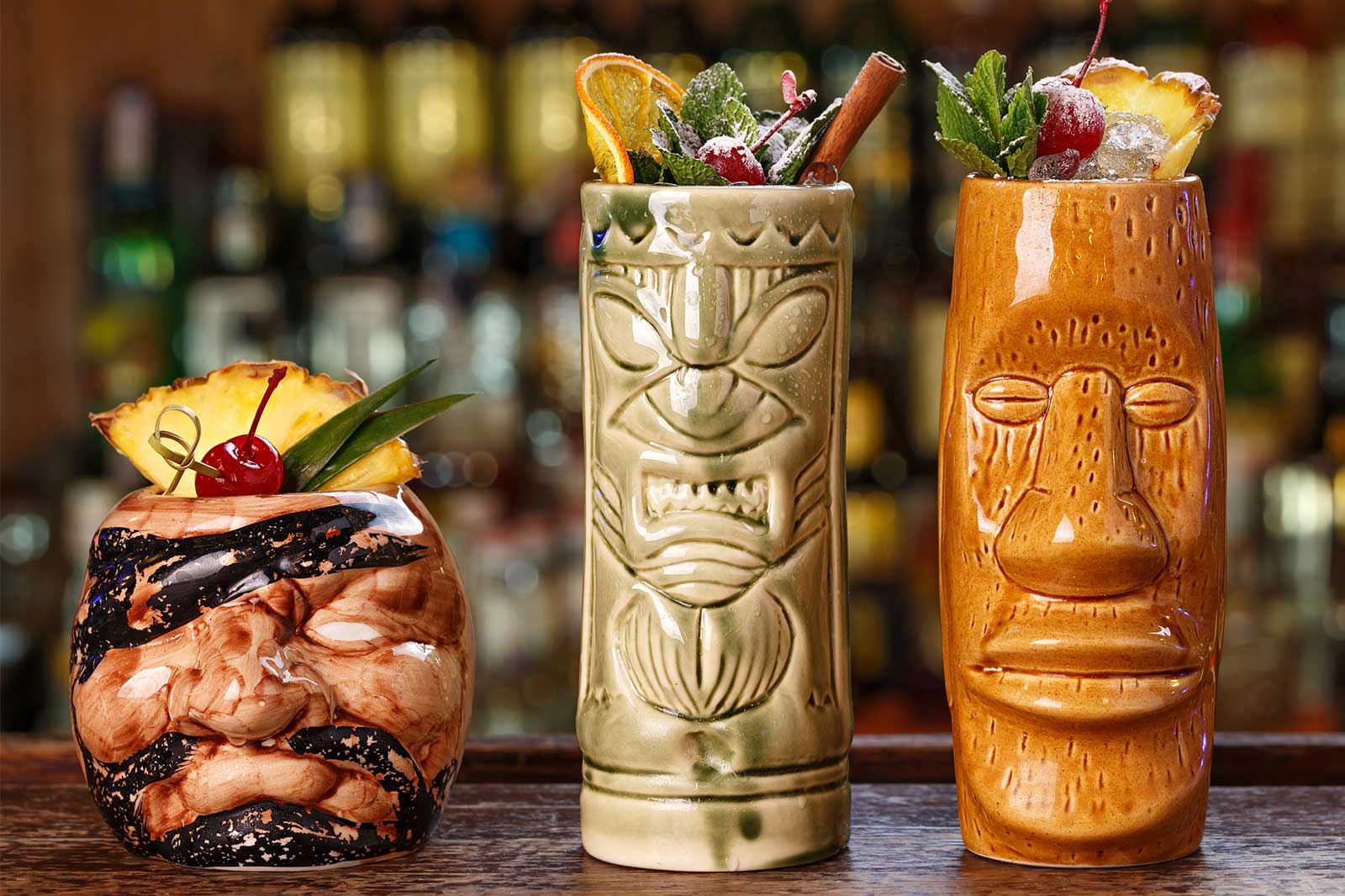The image displays a wooden bar countertop with three tropical tiki-style cocktails in unique, handmade cups. The drink on the left is served in a shorter cup that resembles a deformed pirate face, complete with a beard, mustache, and an eye patch over one eye. It is garnished with a pineapple slice, a cherry, and a couple of leaves. The centered cocktail is in a light gray cup adorned with an orange slice, mint leaves, a cherry, and a straw, along with a sprinkle of white powder on top. The drink on the right, in a brown cup featuring a large face, contains similar garnishes of a pineapple slice, cherries, and mint leaves, but has no straw or cinnamon stick. Behind the cocktails, the background is blurred, showcasing rows of colorful liquor bottles and lights, enhancing the vibrant and festive atmosphere.